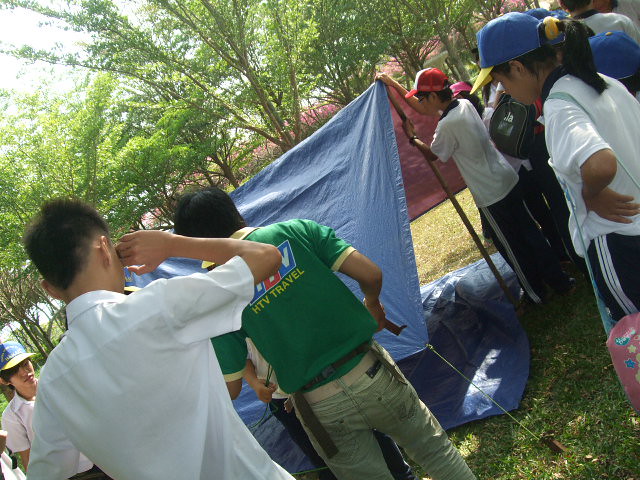In a serene park setting filled with lush green grass and tall trees, a group of about six individuals, primarily of Asian descent, are engaged in assembling a makeshift tent. The tent, crafted from blue tarps, features one man holding up a tent pole to stabilize it. This man stands out with his red hat, white shirt, and track pants. The blue tarps are laid out on the grass beneath, possibly creating a base for sleeping quarters. Around him, various onlookers observe the process of pitching the tent, including a woman with a blue hat and a man clad in a green collared shirt that reads "HTV Travel". The scene evokes a sense of camaraderie, likely indicative of a company outing or team-building event. Additionally, the background is adorned with tall green trees interspersed with pretty pink blossoms, adding to the tranquil atmosphere.